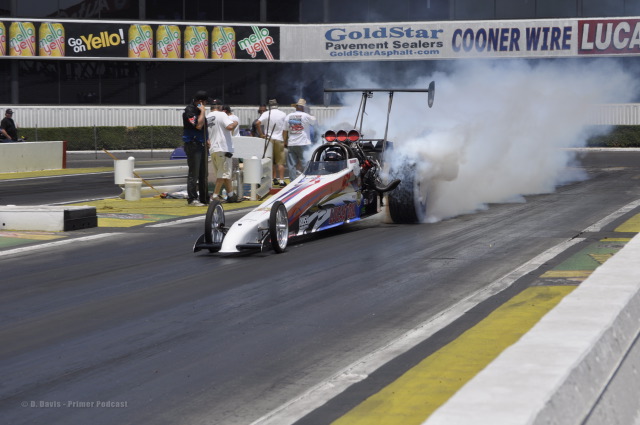The image depicts a dynamic scene on a racetrack featuring a distinctive race car, characterized by its elongated front with skinny wheels and significantly larger rear wheels. The race car, which appears to be captured either at the start or end of a high-speed action, is generating thick clouds of white smoke from its rear tires. The single white car has a bubble compartment occupied by a driver wearing a black helmet. Positioned to the left of the car, a small pit crew of approximately six individuals is standing on the grass, including two men in black shirts and the others in white t-shirts, all wearing hats. There are no other cars visible on the racetrack. In the background, a wall adorned with numerous advertisement banners can be seen, featuring prominent brands such as Mello Yello with the slogan "Go on Yellow," Gold Star Pavement Sealers, and Cooner Wire. The camera angle focuses slightly down the road and tilts to the left. The backdrop of advertising and the dramatic smoke add a vivid sense of action and atmosphere to the scene.